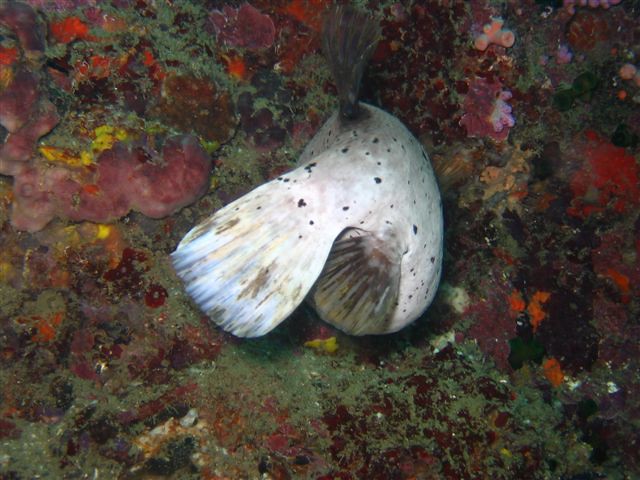The photograph captures an underwater scene centered on a white, spotted puffer fish. The fish is swimming into a small crevice within a coral reef, its tail fin adorned with blue accents facing the viewer, while its dark brown side fins are partially visible. Surrounding the fish, the coral displays a vibrant array of colors, including shades of green, pink, yellow, red, orange, and deep purple. The detailed coral environment also features various plants and algae, adding to the richness of the underwater landscape. The overall scene suggests the fish is seeking shelter or exploring for food within the intricate coral formations.